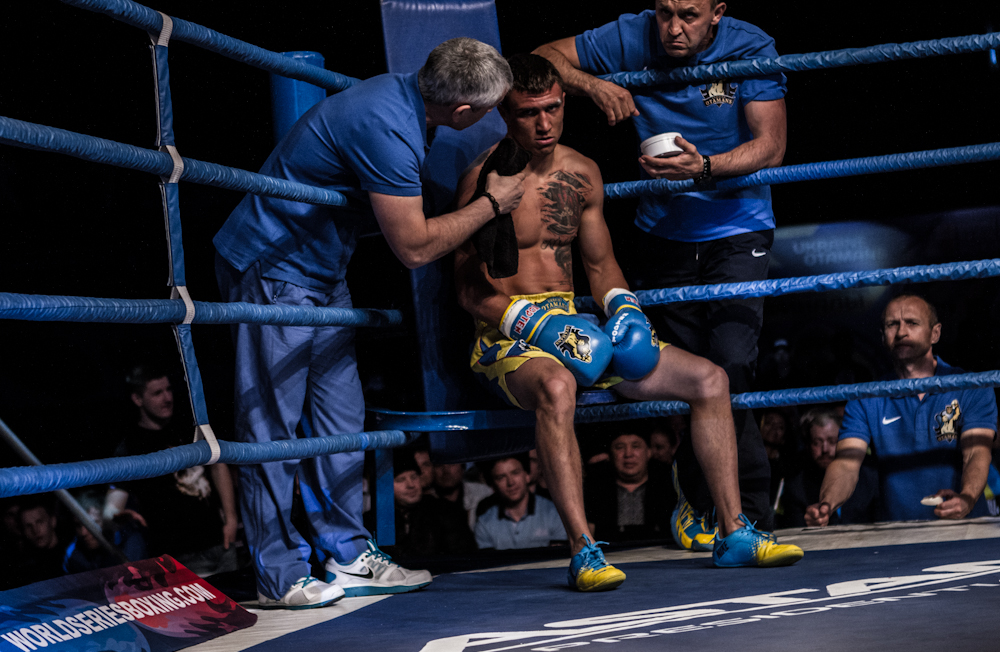The photograph captures a poignant moment in a boxing ring where a weary boxer, sporting a large chest tattoo, sits in the corner between rounds. Wearing predominantly yellow shorts with blue accents, bright turquoise and yellow sneakers, and sky blue boxing gloves, he leans against the blue ropes, emanating exhaustion and intense focus. Two coaches attend to him—one on the left, dressed in an all-blue outfit, speaks intently, possibly giving strategic advice, while the other on the right holds a bowl, possibly tending to his wounds. Behind them, the dimly lit audience watches, adding a dramatic backdrop to the scene. A website, WorldSeriesBoxing.com, is displayed at the bottom left, linking to the event coverage. The blue-dominated ring, complete with blue seats and blue mat, further enhances the atmosphere of this intense moment in the sport.